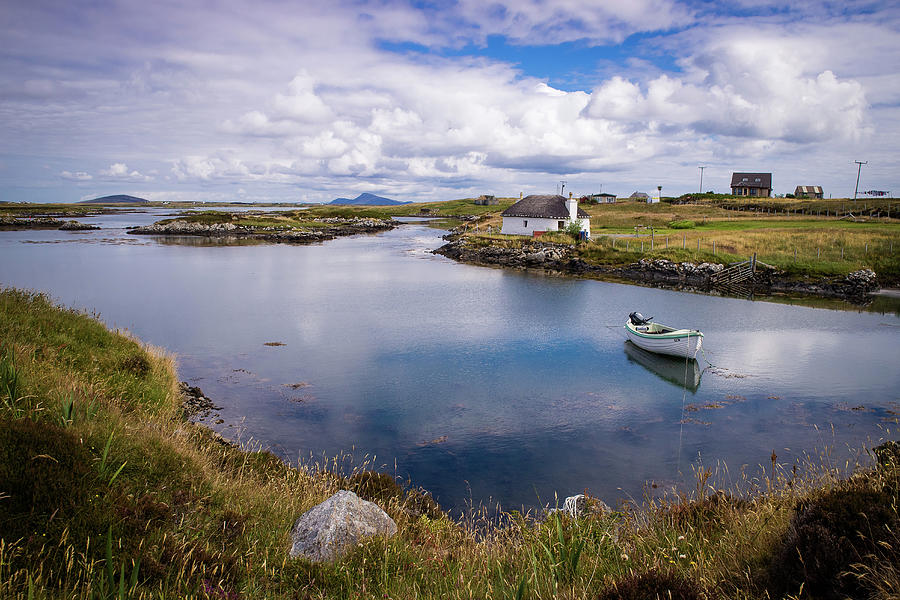The photo captures a serene and picturesque scene of an inlet in the Outer Hebrides of Scotland. In the foreground, a small wooden boat with a distinctive white hull and green trim is tied to the shore with a thin rope. The boat features an oar at the back and a small black and gray outboard motor. The clear waters of the inlet are flanked by rocky banks adorned with patches of grasses and vibrant flowers, creating a beautiful natural setting.

A rustic, rock-built structure with a thatched-like roof stands near the water's edge. This building, possibly abandoned, adds to the quaint charm of the scene. Further back, a story-and-a-half white house with a brick roof and a white chimney can be seen, hinting at nearby habitation despite the absence of people in the image. Beside it, there is a tan and brown barn, and in the distance, another tall, light tan two-story house and several power poles are visible, standing against a backdrop of high, distant mountains.

The sky above is a mix of blue and impressive thunderhead clouds, with the sun peeking through intermittently. This partly sunny weather casts a gentle light over the tranquil seascape, enhancing the natural beauty of the Outer Hebrides inlet depicted in this detailed and atmospheric photograph.